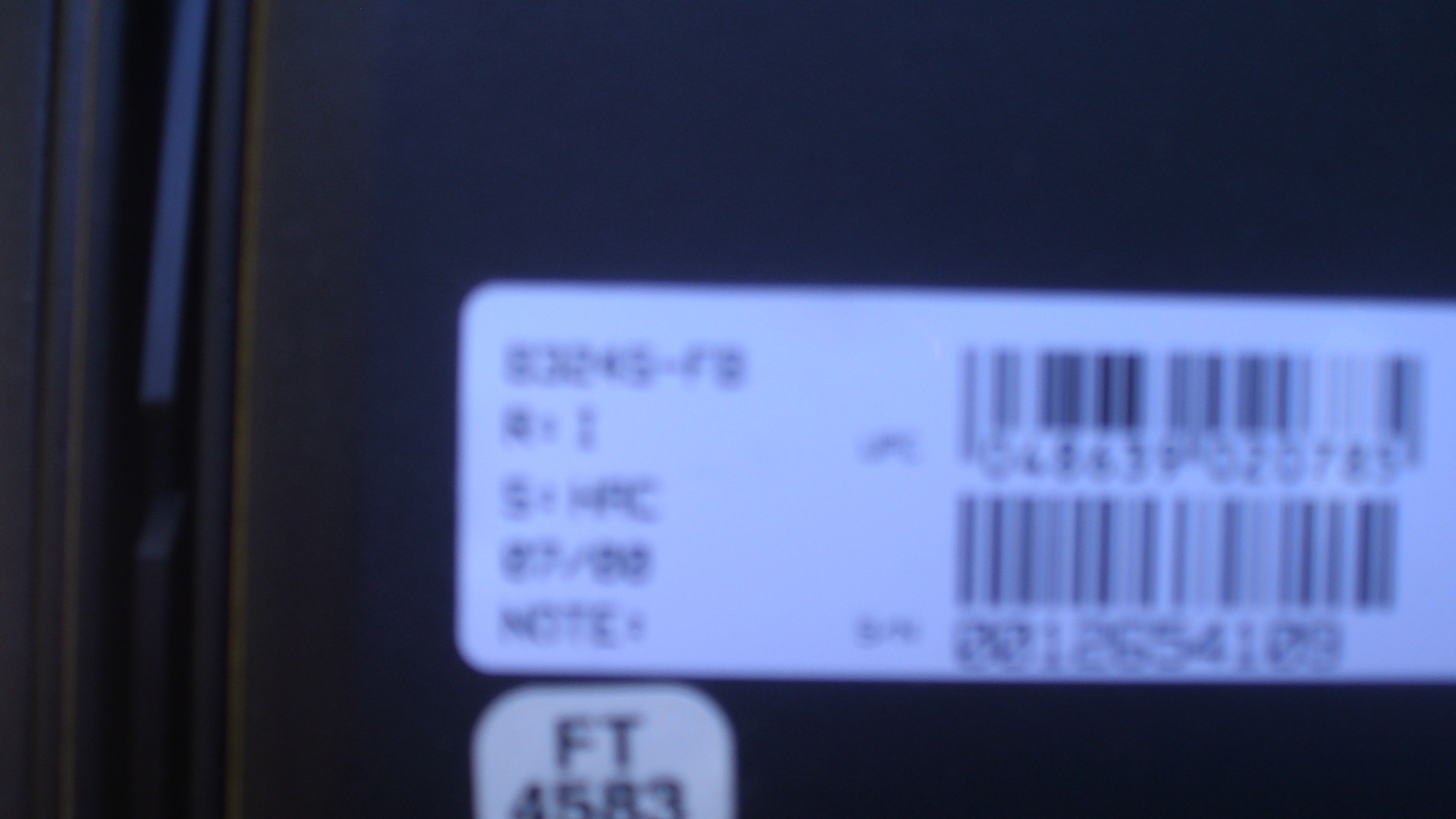The image presents an extreme close-up of a rectangular white label with black text and two black barcodes on a brown object, possibly a piece of furniture or another item. The label's text and barcodes are very blurry, making the numbers and letters difficult to discern. Some black text lines on the left side of the label are particularly illegible. The right side of the label features two distinct barcodes: the top barcode is smaller with a row of numbers beneath it, and a larger barcode is placed below with longer vertical lines and another row of numbers, both of which are unreadable. Below these barcodes is a smaller, square-shaped white label with "FT" at the top and the partially obscured numbers "4583." The brown background shows potential leather-like material with what appears to be a metallic piece on the left side, and further left, another part of the brown item is visible, creating a slight gap.